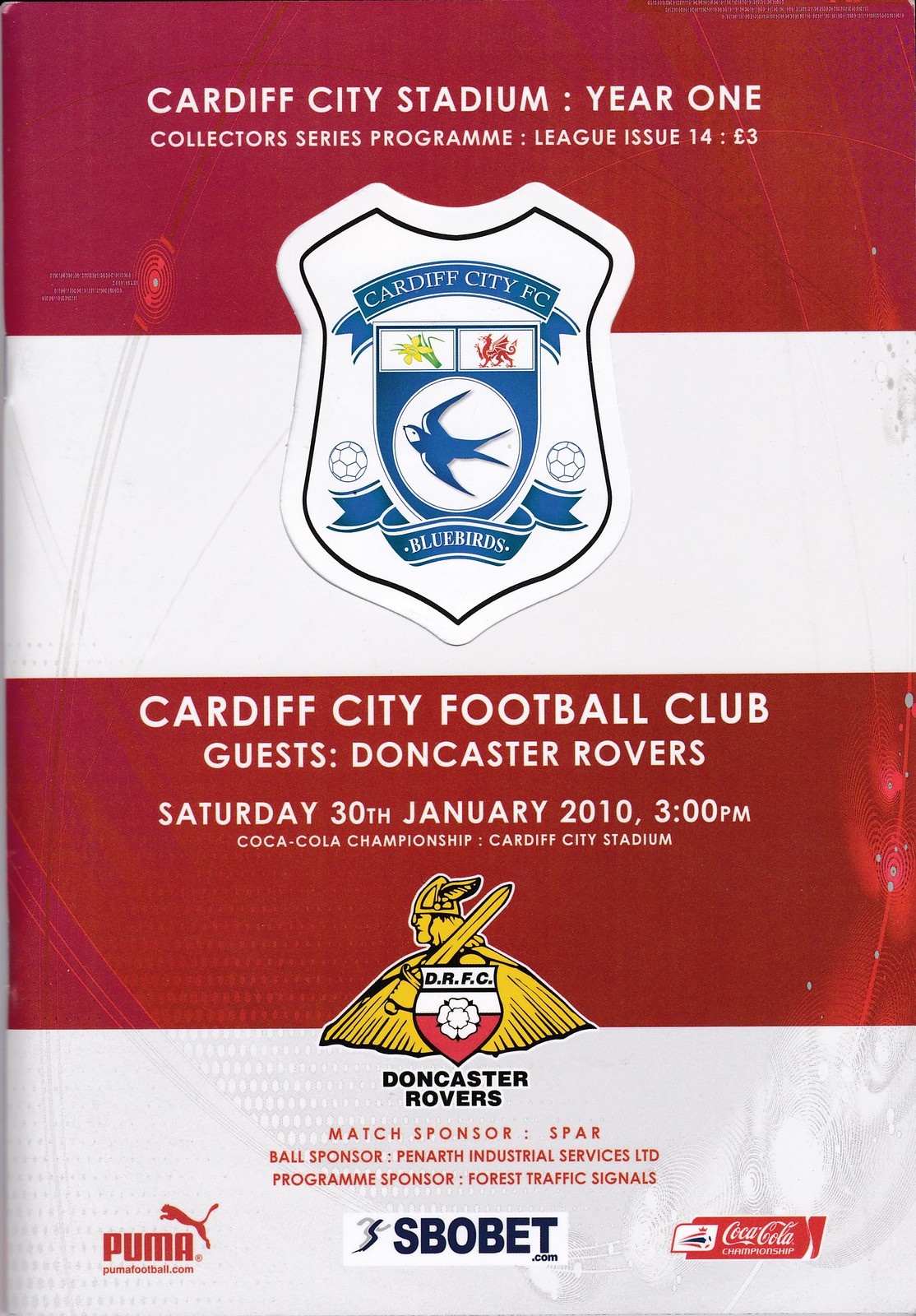The image depicts a crinkled, red and white horizontally striped program cover for a soccer match held at the Cardiff City Stadium. At the top in white text over a red band, it prominently reads: "Cardiff City Stadium: Year One". Below, in smaller type, it continues: "Collector Series Program: League Issue 14: 3 Pounds". Situated beneath this, a white shield logo features a bluebird with a banner that reads "Bluebirds", flanked by a daffodil-like flower, a griffin, and two soccer balls. In the red band below, white text states: "Cardiff City Football Club Guests Doncaster Rovers, Saturday 30th January 2010, 3 p.m.". Further down, a gold emblem showcases a figure wearing a Viking hat with wings and holding a sword, labeled "Doncaster Rovers". The bottom portion of the cover includes small sponsor logos, featuring brands like Puma and Coca-Cola. The overall design is rich in detail, presenting a comprehensive, textured visual of this collector's series soccer program.